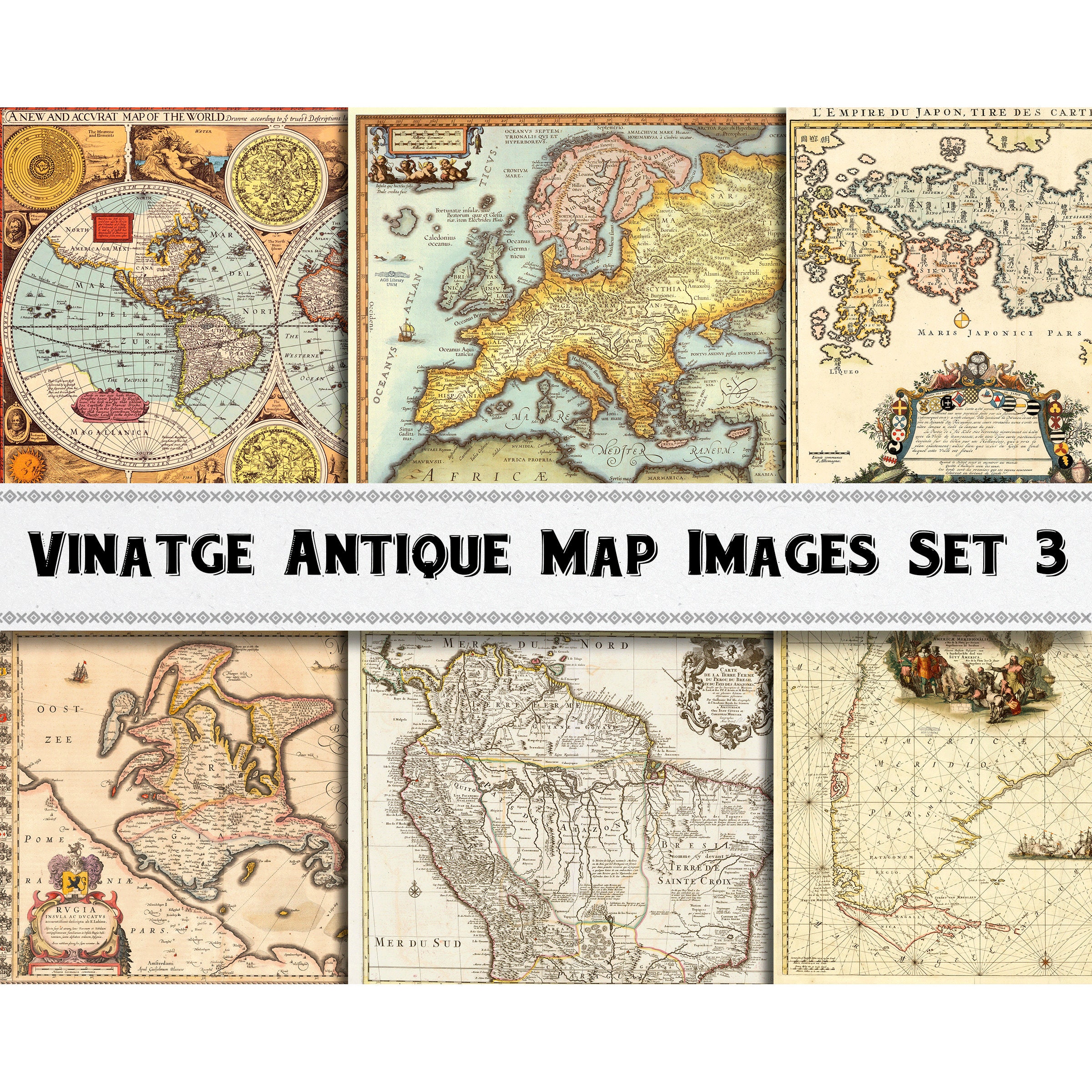The image features six distinct, well-preserved antique maps arranged in two rows of three. Each map appears crisp and meticulously detailed, indicative of high-quality reproductions. At the center of the image, a white rectangle with an X and diamond pattern in gray adorns the top and bottom edges, housing bold, capitalized black text that reads "Vintage Antique Map Images, Set 3."

In the top row, the leftmost map depicts the entire globe. The central map appears to be an ancient representation of Africa, possibly encompassing parts of Europe as it is labeled with "Ocean’s Atlantic." On the far right, the map is titled "Empire du Japan," clearly illustrating the old Japanese Empire.

The bottom row contains three more maps of similar antique style, their pristine condition highlighting the attention to detail in these reproductions. The overall presentation is bright and clear, allowing for an unobstructed view of each map's intricate design and layout.